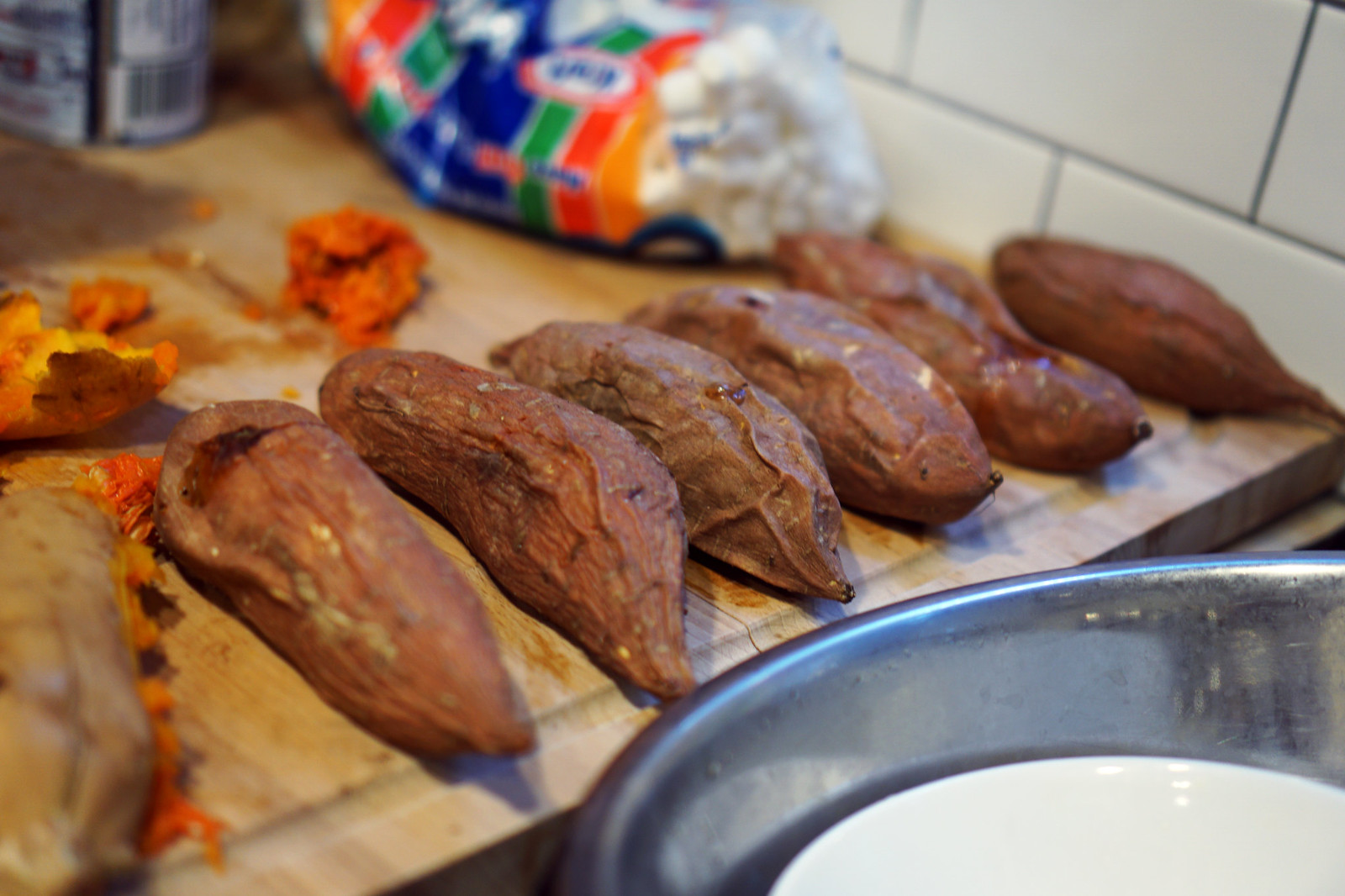This image captures a detailed kitchen scene with a white tiled wall as the backdrop. On a wooden cutting board situated on a counter, there are seven roasted sweet potatoes, with one cut open to reveal its vibrant orange flesh. The sweet potatoes are well-cooked, showcasing crispy, wrinkled skins with some of their juices visibly oozing out. Towards the back, a piece of sweet potato appears smashed, leaving a reddish blob. Dominating the center of the cutting board is a plastic bag of mini marshmallows, branded likely under Kraft, characterized by horizontal blue, green, orange, and red stripes, though the brand name is somewhat illegible. Tiny white marshmallows peek through the bag. In the foreground, a stainless steel bowl with a smaller white glass bowl inside adds to the complex arrangement, hinting at preparations for a dish possibly involving candied sweet potatoes.